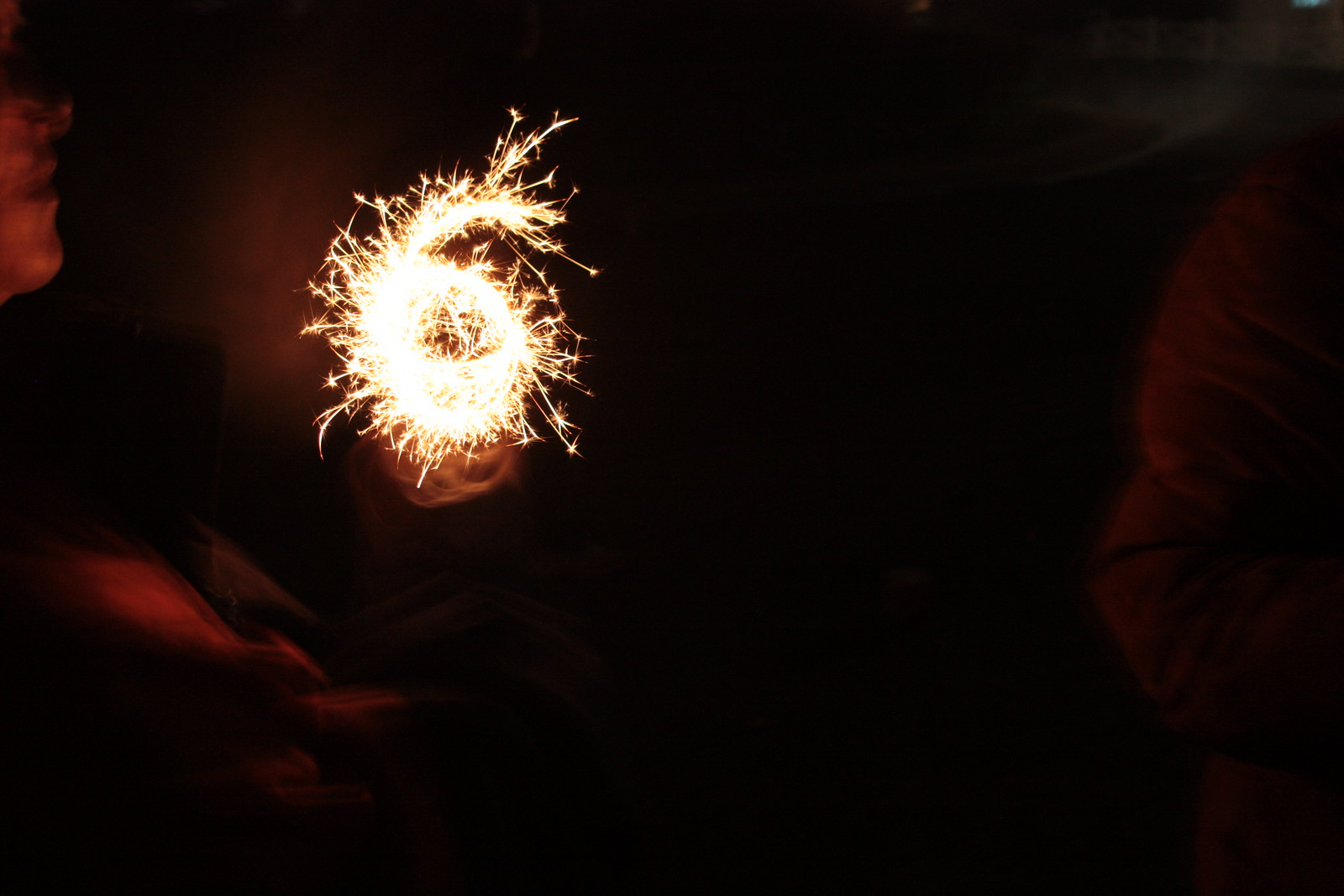In this captivating nighttime photograph, a dazzling sparkler illuminates the darkness with its swirling trail of burning embers. Positioned in the top left corner, the sparkler's motion creates a distinct number six, leaving a luminous yellowish-white glow amidst the predominantly black background. The long exposure captures the dynamic movement, resulting in a slightly blurred image that conveys a sense of motion.

On the left side, the faint, double-exposed side silhouette of a person's face emerges, their features softly lit by the sparkler's glow. The blur adds a dreamlike, ethereal quality to the scene. Just below the sparkler, one can vaguely discern the shape of a hand, suggesting that the person is holding the sparkler. Additionally, a faint dark brown outline on the right side hints at another person's clothing, though its indistinct form adds to the mysterious atmosphere of the image.